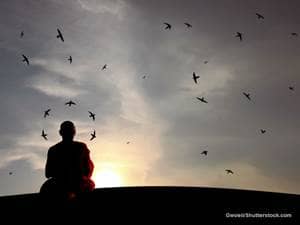This detailed photograph portrays a serene sunset scene characterized by the silhouette of a monk in prayer, situated in the lower left-hand corner. The image's depth is enhanced by the dark silhouette of the earth at the bottom, melding seamlessly into the monk's figure, which is primarily depicted in black shadow. However, a subtle glimpse of a red cloak can be discerned on his right side.

The sunset, positioned just to the right of the monk, casts a brilliant white-yellow glow, surrounded by an orange hue that fades into the deep gray and white clouds above. This dramatic transition in the sky's colors beautifully contrasts with the stark blackness of the ground and silhouette.

A striking feature of the photograph is the formation of five birds, perfectly aligned around the monk's head, forming a quasi-three-quarter circle. Each bird is equidistant from his head, enhancing the ethereal aura surrounding his silhouette. Additional birds are scattered throughout the sky, adding to the natural ambiance of the scene.

In the lower right corner, there is some white text, although it is too small to be readable. This text, along with the image's compact dimensions—approximately two inches wide and an inch and a half high—suggests an intimate, carefully composed snapshot that conveys a moment of peaceful reflection.